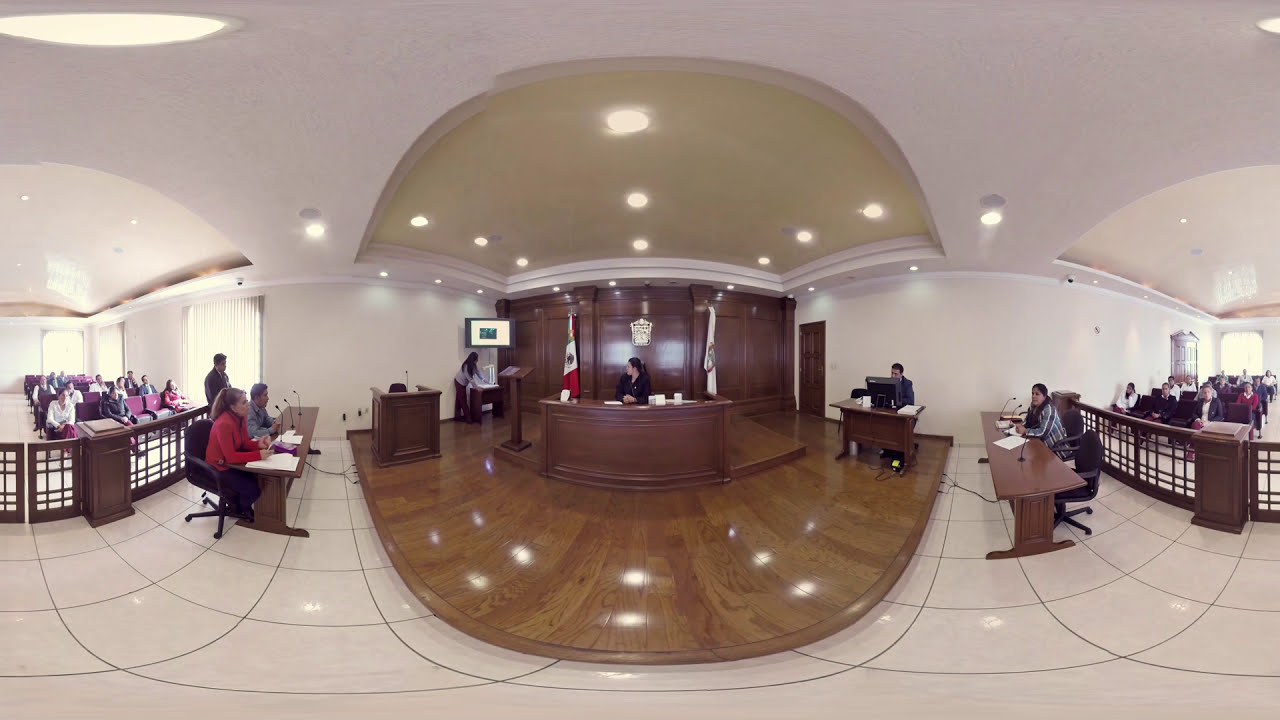The photo captures an indoor scene of a courtroom in Mexico, identified by the presence of a Mexican flag near the judge who is central to the image, seated at a wooden desk. The judge, wearing a black robe, commands the focal point of the room, flanked by two flags, one on either side. On the left and right of the judge's desk are two wooden tables, where lawyers are seated with microphones in front of them, suggesting the presence of both the plaintiff and the defendant. Positioned on the right side is a man working on a computer, likely the record keeper. In front of the judge’s desk are two chairs, possibly for witnesses. The courtroom has a white-tiled floor, and behind wooden barriers on both sides, a crowd sits attentively, indicating public attendance during the proceedings. The entire scene is illuminated with overhead lights, contributing to a formal ambiance.